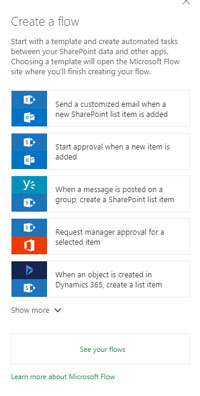Here is a cleaned-up and detailed version of the image caption:

---

The image depicts a screenshot from a website featuring text against a white background. At the top of the page, in a larger font size, the title "Create a Flow" is prominently displayed, with the letter 'C' capitalized. Above this title, on the right side, there's an upward-pointing arrow icon.

Beneath the "Create a Flow" title, the text reads: "Start with a template and create automated tasks between your SharePoint data and other apps. Choosing a template will take you to the Microsoft Flow site where you'll finish creating your flow." The term "SharePoint" is written with a capital 'S' and a capital 'P'.

Proceeding downward, the page is divided into five square sections, each representing different templates with associated graphics:

1. **Template 1:** A blue background, with the graphic indicating a customized email. The text reads: "Send a customized email when a new SharePoint list item is added."
2. **Template 2:** Another blue background similar to the first one, with graphics suggesting an approval process. The text states: "Start approval when a new item is added."
3. **Template 3:** Split into two colors, teal on the top half and a greenish-blue on the bottom half. It reads: "When a message is posted on a group, create a SharePoint list item."
4. **Template 4:** Also divided into two sections, with blue on top and red on the bottom. The text here is: "Request manager approval for a selected item."
5. **Template 5:** Featuring a navy top half and a blue bottom half, this square says: "When an object is created in Dynamics 365, create a list item."

Below these template squares, text says "Show more" accompanied by a downward-pointing arrow.

At the bottom of the image, two lines of green text appear: "See your flows" followed by "Learn more about Microsoft Flow."

---

This caption provides a detailed and structured description of the image, ensuring clarity and a better understanding of its contents.